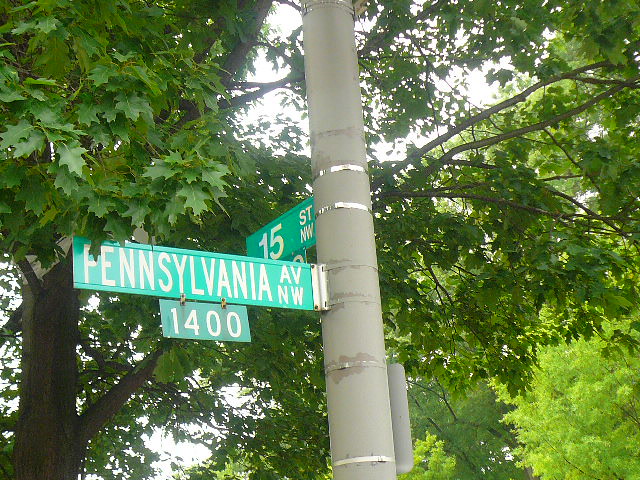This photograph captures an outdoor scene featuring a symphony of verdant foliage and urban elements. Dominating the composition are lush trees with leaves ranging from dark to lighter green shades, forming a thick canopy with sporadic gaps revealing an overcast sky, heavy with shades of gray as though heralding or receding from a storm. Centrally framed is a tall, light gray cylindrical pole adorned with silvery rivets that occasionally catch the light. Attached to the pole are multiple green street signs with white text: one sign on the left clearly marking "1400 Pennsylvania Avenue NW," and another indicating "15th Street NW." The intricate play of light and shadow across the leaves and the pole adds depth to the scene, suggesting a serene yet dynamic intersection nestled in a leafy neighborhood.